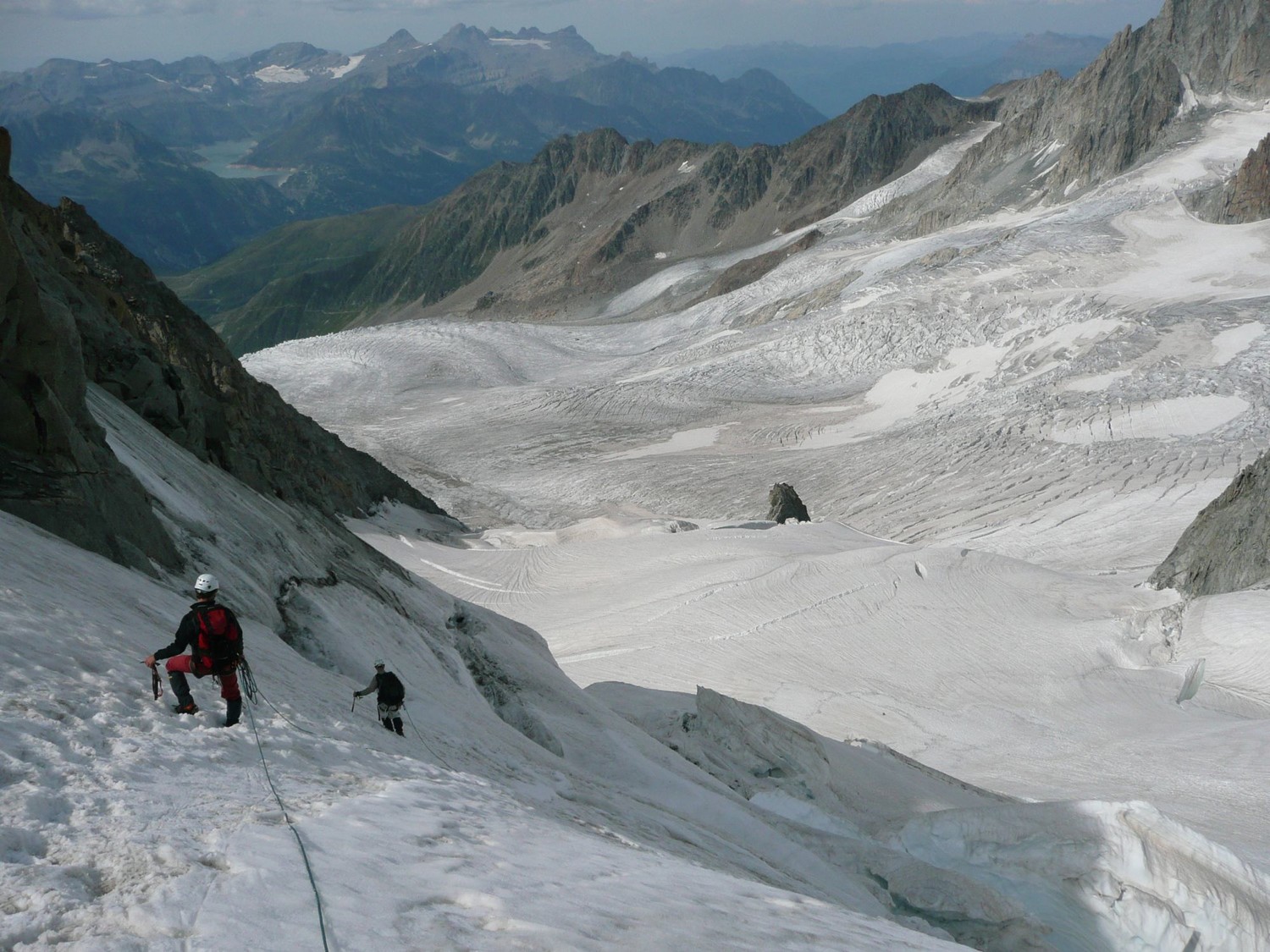The image depicts a rugged, snow-covered mountainous region reminiscent of the Alps, with majestic peaks and glaciers dominating the landscape. At the forefront to the bottom left, a man dressed in a black bodysuit and red vest clings to the side of the mountain, using a rope for support. This rope, essential for his safety, extends downward and attaches to another climber below, who is wearing a similar black bodysuit with light grey pants. Despite the small size of the second climber in the image, his struggle to ascend is evident. Both men are equipped with white helmets and are engaged in a meticulous climb, securing stakes and using their gear to navigate the icy, windblown terrain. The central part of the image reveals a mixture of pristine white snow and dirty, wind-swept patches, while the background fades into a hazy blue mist, accentuating the distant peaks and rugged terrain. The scene is both intense and serene, capturing the harsh beauty of the mountainous adventure.